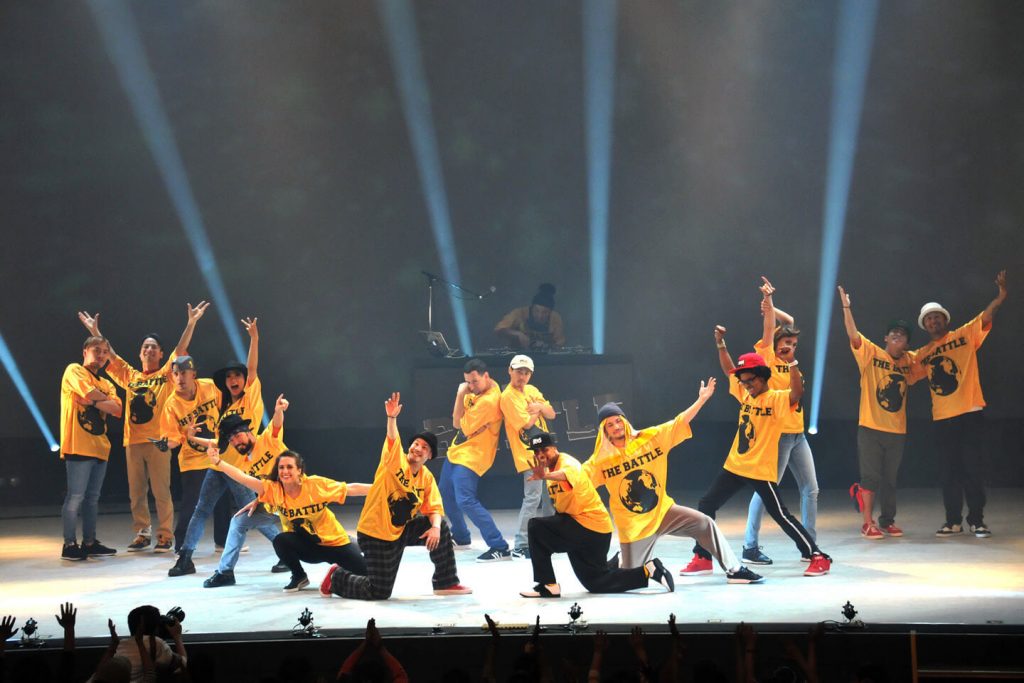In this live concert photograph taken in landscape mode, a vibrant dance troupe of 15 participants occupies a well-lit stage with a white floor set against a dark gray and black background. Illuminated by blue and green lights that stripe vertically, the troupe members wear matching yellow t-shirts emblazoned with the words "The Battle" in black letters, each featuring a black globe graphic. The performers, in a mix of blue and black jeans with a few donning hats, are striking dynamic poses—some standing, others kneeling or with their hands raised, marking the finale of what appears to be an exhilarating rap or breakdancing battle. Behind them, the DJ, faintly visible with a microphone and turntables, adds to the electrifying ambiance. The indistinct hands of an applauding crowd can be seen at the bottom edge of the frame, enhancing the scene's live energy.